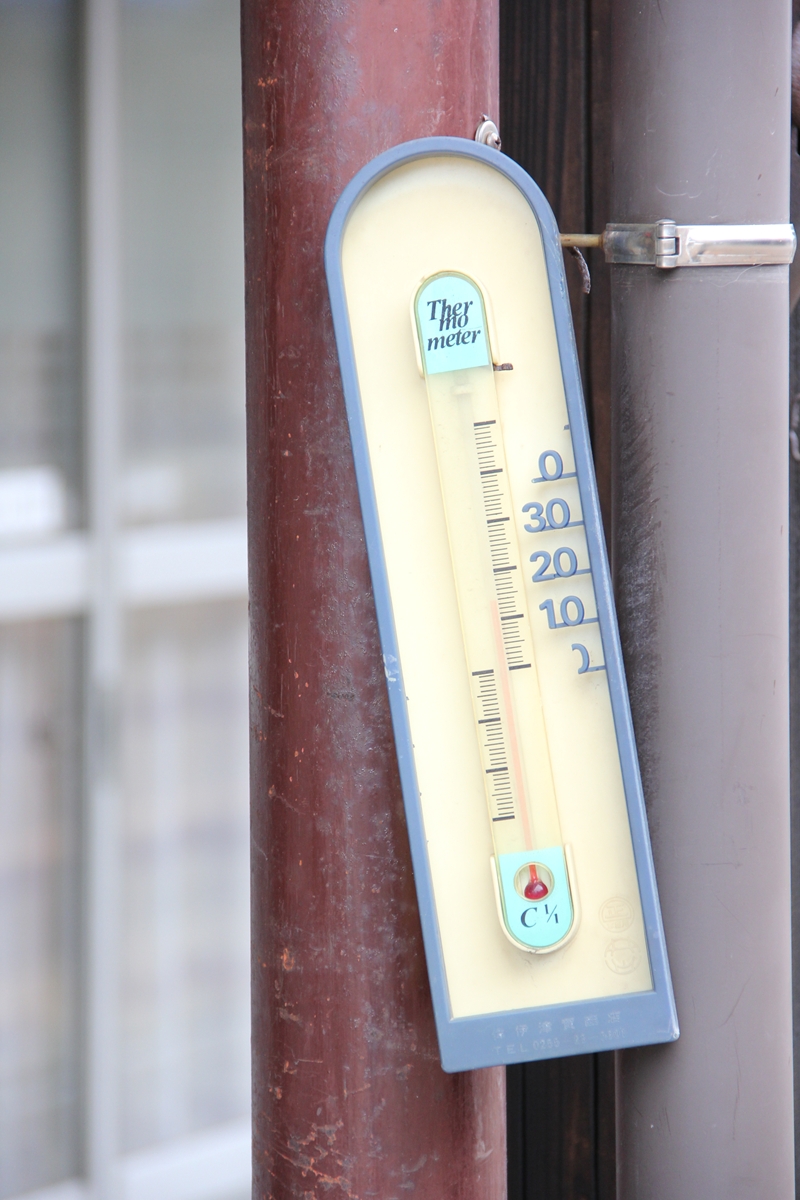This outdoor photograph captures a vintage thermometer fixed to a weathered, rust-colored pole. The thermometer itself features a straight base with a rounded top, emblazoned with the word "THERMOMETER" divided into three rows: "THER," "MO," and "METER." The temperature scale is marked with intervals of 0, 10, 20, and 30 degrees, with additional minor markings and a partially visible half-circle indicative of further measurements. At the bottom of the scale, the notation "C" suggests Celsius, followed by an unclear fractional value. The thermometer's bulb is red, obscuring the current temperature reading. In the background, a gray pole and a window divided into four sections are also visible, reinforcing the outdoor setting.